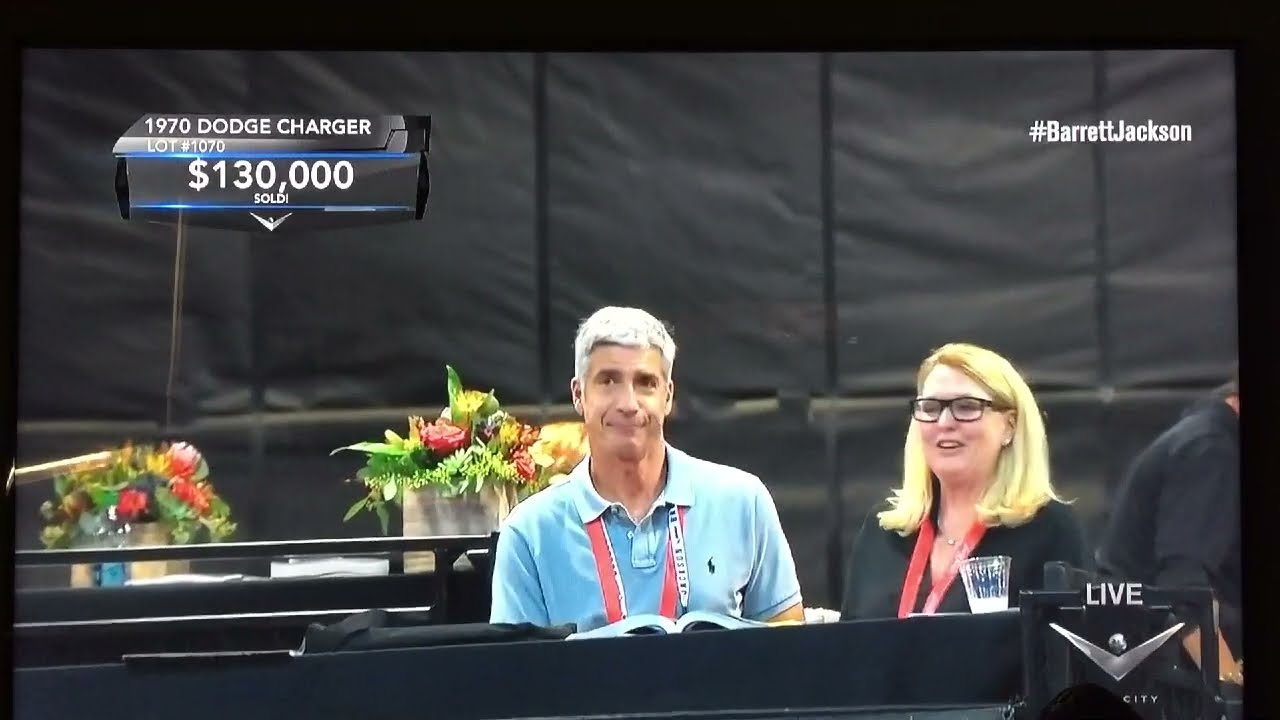In this overexposed and brightly lit image taken in a large showroom, the focal point is a shiny white convertible sports car, possibly an Audi, featuring red leather seats and silver, shiny wheels. The car has its hood up, revealing a polished silver bumper and distinctive bright headlights. Surrounding this car are several other vehicles, including another white car to its right, a blue car to the left, and a couple of red cars blurred in the background. The showroom is populated by a few older men casually standing around, engaging in conversations, with the powerful lights illuminating the scene mainly from the upper left side, leaving the upper right side darker in contrast.